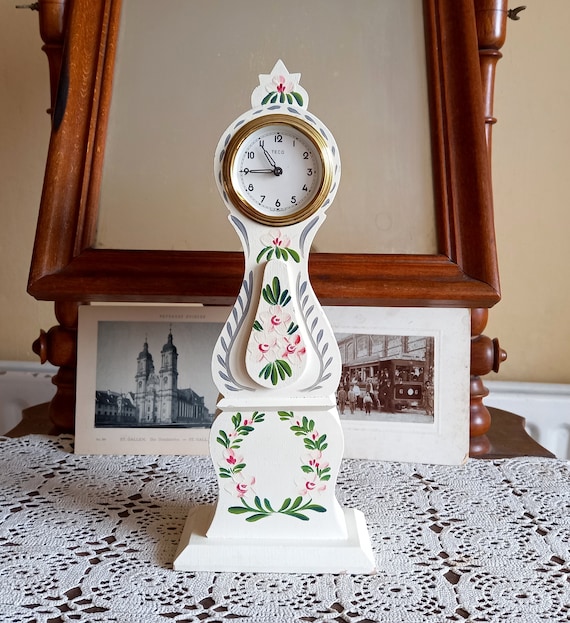The image showcases a unique clock-like structure with vibrant greens, reds, and grays mixed with white oak colors. Positioned centrally is a traditional 12-hour gold-trimmed circular clock displaying the time, adorned with intricate floral designs and pink wreaths. The clock, constructed in a tiered format with a square base, stands elegantly on a detailed white lace doily over a wooden surface. Behind it are two antique black-and-white photographs; one depicts several men preparing to board a public bus, suggesting a scene from over a century ago, possibly from the Victorian era or London. The second photograph shows an older building. These historical photos enhance the vintage feel of the setting. Above them is a tall, wooden-framed object that resembles a mirror but lacks a reflective surface, perhaps functioning as a picture frame. The background includes a beige wall with white wainscoting, adding to the scene’s classic and timeless ambiance.